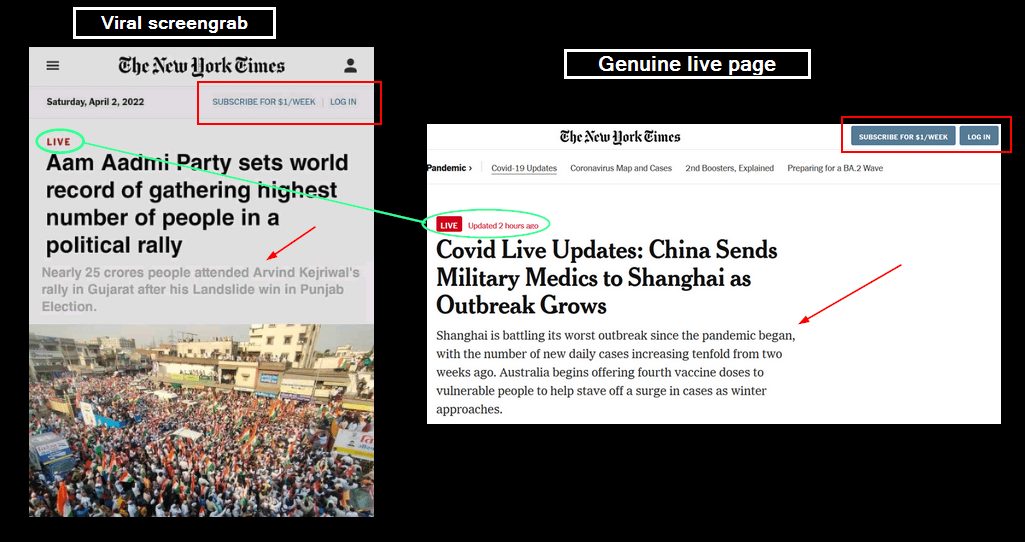**Screenshot of New York Times Articles with Significant Updates**

This screenshot captures two articles from the New York Times, dated Saturday, April 2, 2022. The header of the screenshot prominently displays "Viral Screen Grab" in white font, with "The New York Times" branding visible beneath it. To the left of the header is a menu button, and to the right, a personal sign-on button. The banner also includes a subscription offer that reads, "Subscribe for $1 a week, log in live."

The first highlighted article announces a significant achievement by the Aam Aadmi Party, stating, "Aam Aadmi Party sets world record of gathering highest number of people in a political rally." It details that nearly 25 crores (250 million) people attended Aravind Kejriwal's rally in Jakarta following a landslide victory in the Punjab election.

Adjacent to this, the second featured article provides a "COVID Live Update." It reports on China's response to a severe COVID-19 outbreak in Shanghai, noting that military medics have been deployed as the number of new daily cases has surged tenfold over the past two weeks. Additionally, it highlights that Australia has begun offering fourth vaccine doses to vulnerable populations to mitigate a potential rise in cases as winter approaches.